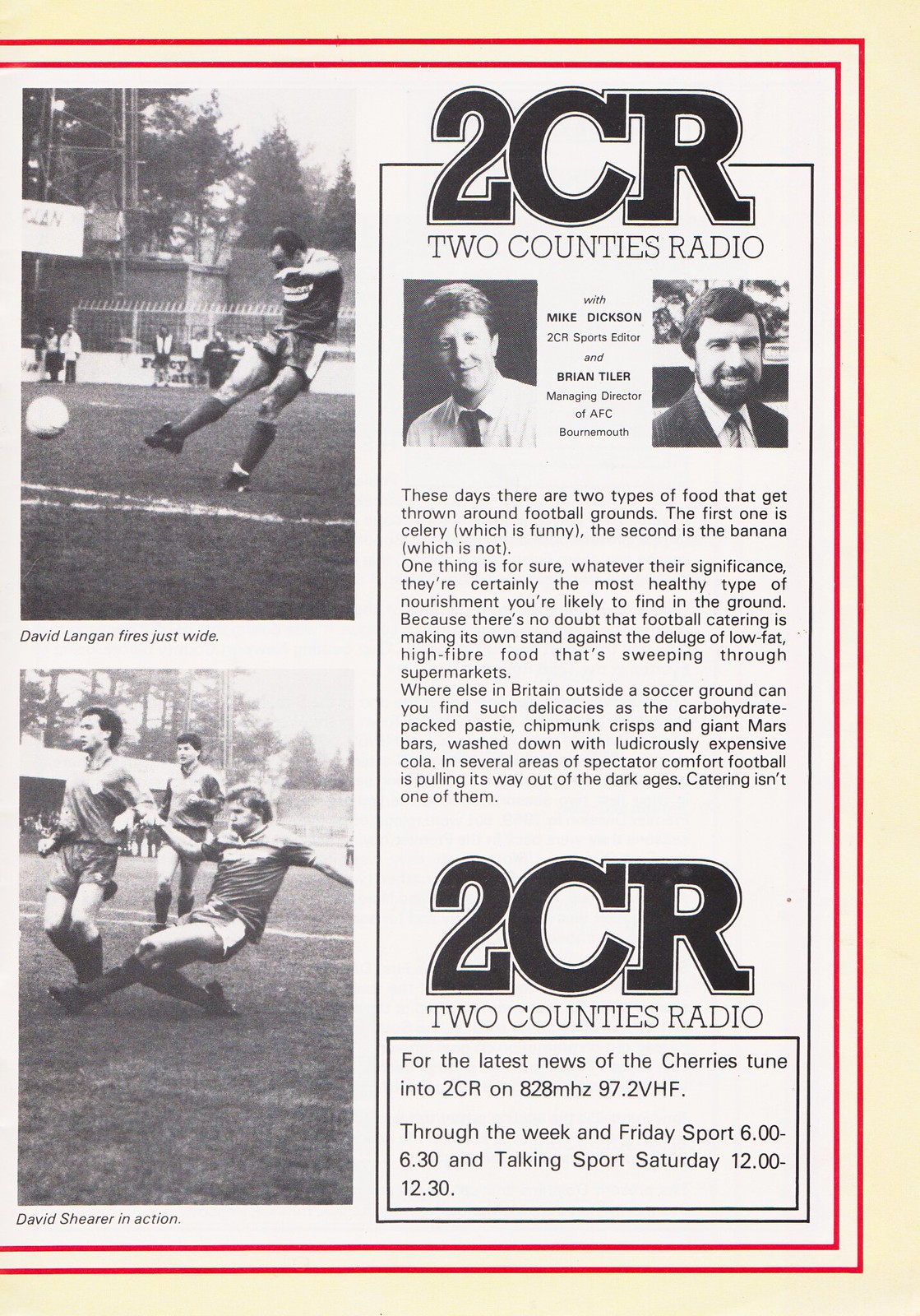This image is a clipping from an old black-and-white newspaper or magazine article, featuring a detailed layout with photos and text. The overall article is bordered in red, and the content sits against a white background. On the left side are two black-and-white photos from a football match. The top photo captures David Langan in mid-action, having just kicked a soccer ball with significant force, his body leaning back and his left arm extended forward as he looks down at the ball. Below this, another photograph shows a sequence of three players in motion: one player appears to be sliding and close to falling, having likely just kicked the ball, while the other two players watch its trajectory. Accompanying captions identify the players as David Langan and David Shearer, respectively.

On the right side of the clipping, a bold, large heading "2CR" is prominently displayed, referring to "Two Counties Radio." Below this, two hosts are pictured: Mike Dixon, the 2CR Sports Editor, and Brian Tiller, the Managing Director of AFC Bournemouth. Dixon, clad in a white shirt and black tie, faces Shearer, who is dressed in a black suit with a white shirt and black tie, sporting short hair and a beard. Accompanying the images is a dense text article discussing the peculiarities of stadium food, noting the amusing presence of celery and bananas and contrasting them with the typical offerings of pasties, crisps, and Mars bars. The article critiques the outdated nature of football catering in comparison to other improvements in stadium amenities.

Further information about the 2CR radio programs is provided at the bottom of the article, listing the latest sports news available on 828 megahertz, 97.2 VHF. It mentions specific program times, including Friday Sports from 6 to 6:30 PM and Talking Sports on Saturday from 12 to 12:30 PM.